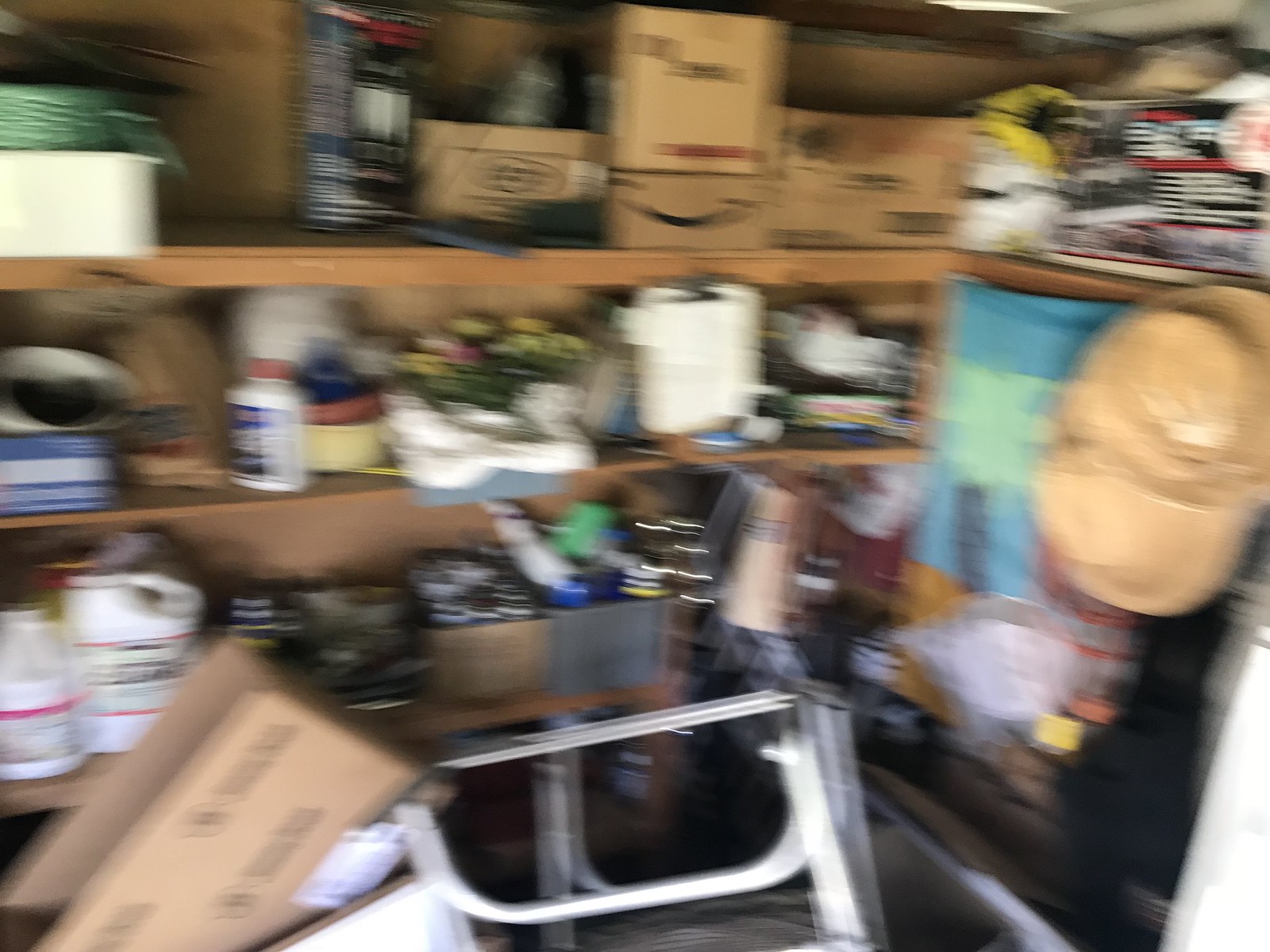The image depicts a cluttered garage interior, characterized by its blurry quality. Dominating the scene is a large rectangular shelving unit with multiple open wooden shelves. The shelves, at least three in number, are filled chaotically with various items. Beneath the bottom shelf, additional objects are stacked. The items range from Amazon-style brown boxes to retail packaging in black and red colors. Among the assorted contents, there are what appear to be hats, a towel, tools, rolls of paper towels, and jugs possibly containing ant spray or poison. The overall impression is one of disarray, with numerous household and garage items crammed together, making it difficult to discern specific objects due to the image's blurriness.